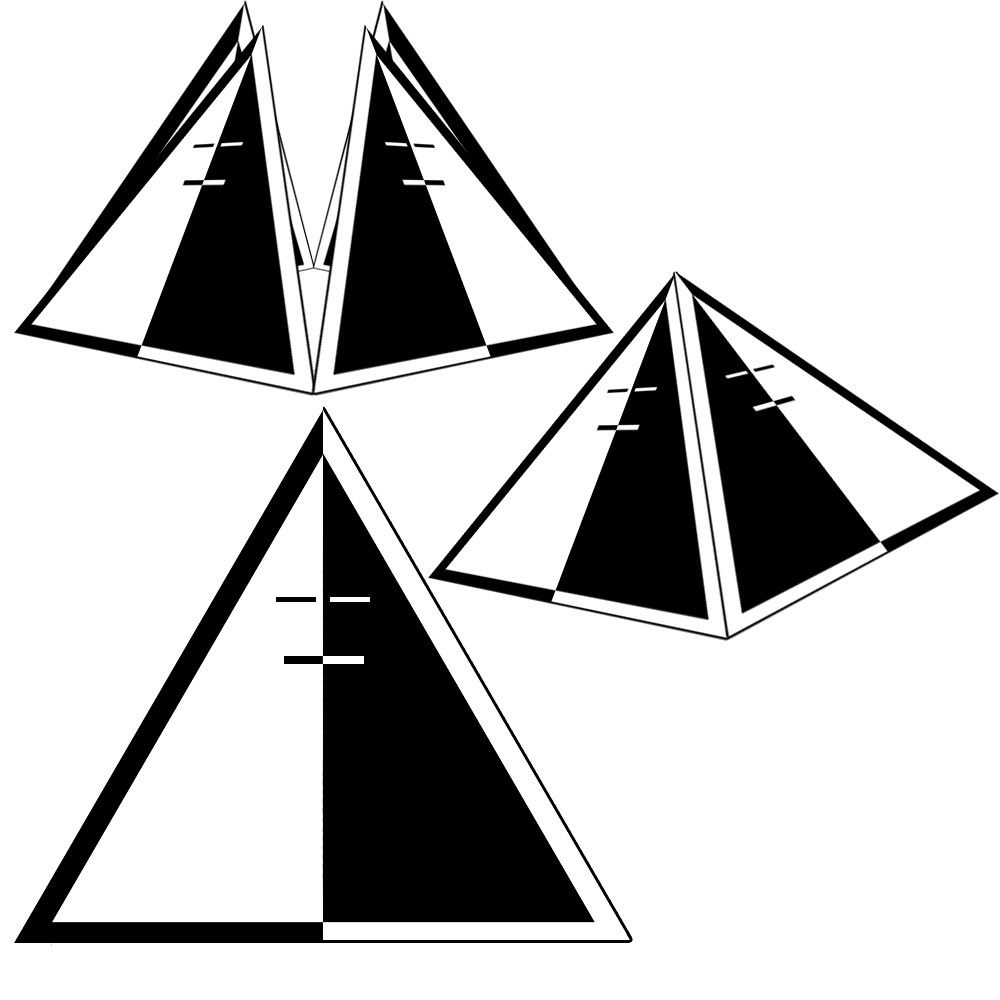The image depicts a step-by-step diagram on a white background, illustrating a black and white geometric structure that resembles an origami game or a 3D pyramid. At the bottom left of the image, there is a single triangle divided into two halves: one half black and the other half white. This triangle has contrasting edges where the black half has a white edge and the white half has a black edge, and features four lines that extend across it, matching the background color.

To the upper left of this triangle, there appears to be an "opened" structure showing four distinct triangular panels, each alternating in black and white, suggesting the makeup of a more complex shape when combined. 

On the right side, a fully formed 3D pyramid constructed from these alternating black and white triangles is shown. This arrangement gives the visual impression of parts falling together to form a complete triangular pyramid.

Overall, the illustration combines three views: a single, detailed triangle; an exploded view of four triangular components; and a complete 3D pyramid showcasing the intricate design of black and white geometrical shapes.